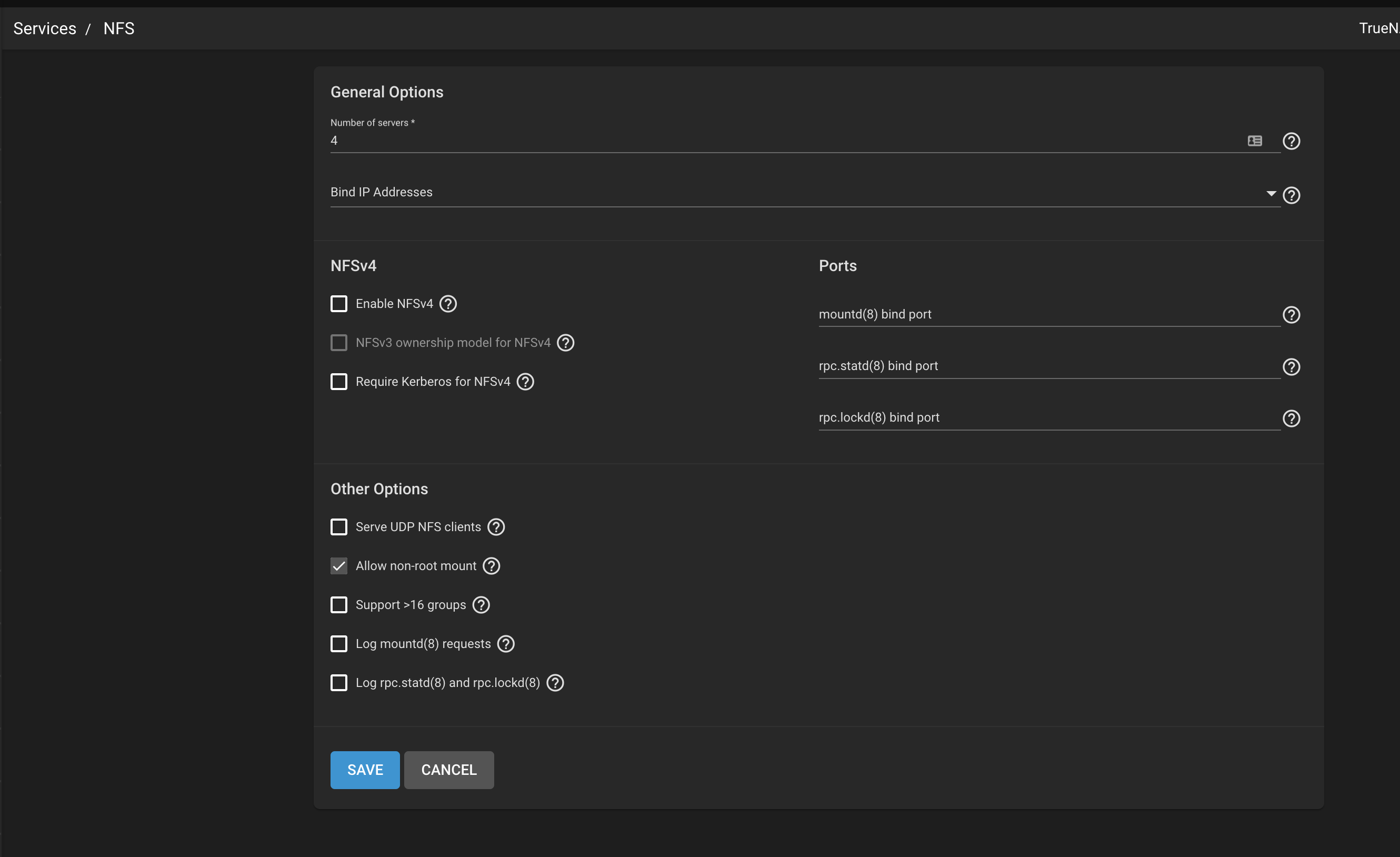In this detailed image of a website interface, we are currently navigating the "Services" section, specifically on the NFS (Network File System) page, as indicated by the path "Services/NFS" located at the top left corner. The layout is as follows:

**General Options:** 
- There is a drop-down menu labeled “Number of servers,” with the current selection set to 4.
- Another drop-down menu labeled “Bind IP addresses” remains unselected.

**NFS v4 Options:**
- A title labeled “NFS v4” is present beneath the general options.
- Three checkboxes are listed under this category:
  1. **Enable NFS v4:** Accompanied by a question mark icon, which likely provides additional information about NFS v4. This option is currently unchecked but can be enabled.
  2. **NFS v3 Ownership Model for NFS v4:** This option is grayed out and marked with a question mark for further details, suggesting it is inactive or unavailable for selection.
  3. **Require Kerberos for NFS v4:** 
   
**Port Options:**
- To the right, there is a section labeled “Ports,” with specific fields for:
  - Mount bind port
  - RPC statd bind port
  - RPC lockd bind port

**Other Options:**
- The section titled "Other Options" includes several configurations with checkboxes:
  - Serve UDP NFS clients
  - Allow non-root mount
  - Support less than 16 groups
  - Log mountd requests
  - Log RPC statd 
  - Log RPC lockd
  - Alongside each of these options, question mark icons are available for more information.
  
**Action Buttons:**
- At the bottom of the interface, two buttons are visible for user actions: "Save" and "Cancel".

This interface provides a comprehensive set of configurations for managing NFS services, including server settings, IP binding, NFS version options, port allocations, and various other customizable features.